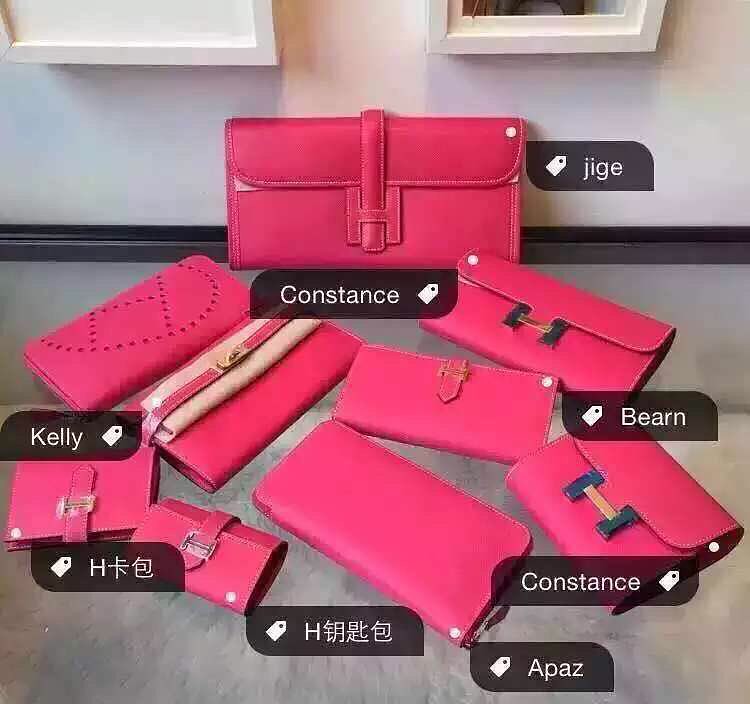The image depicts nine hot pink handbags and wallets arranged on a light gray surface against a white wall. The various styles of purses, including clutches and pocketbooks, are meticulously organized in a way that showcases their diverse designs and sizes. Each item is labeled with a small dark gray or black rectangular tag featuring names such as “JIGE,” “Constance,” “Bearn,” “Constance,” “Apaz,” two labels in non-English (Asian) characters, and “Kelly.” The purses exhibit different fastening mechanisms including clasps, zippers, buckles, and snaps, with some showcasing intricate stitching and designs. The background includes glimpses of two framed pictures, visible only by their bottom edges, further drawing attention to the collection of vividly colored accessories.